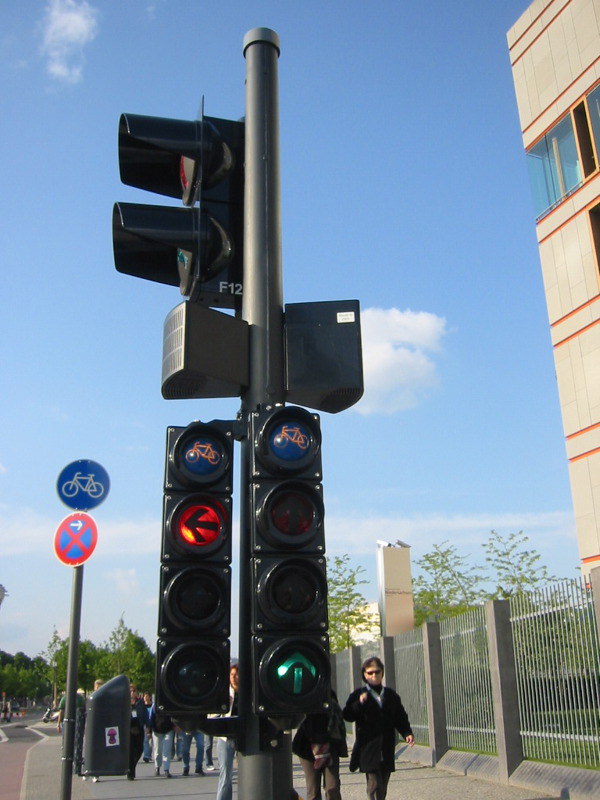This vivid color photograph captures a lively urban scene on a bright, sunny day with a clear blue sky and a few wispy clouds. Dominating the foreground is a tall, thin black traffic light pole extending from the bottom center to the middle of the image. The traffic light has four signals; the front-facing portion displays a lit red arrow pointing left and a green arrow pointing up. Below these arrows is blue signage with bicycles, and another sign with a blue circle and red X beneath it.

In the background, a tan building with orange trimming stands prominently to the right-hand side, partially obscured by a high black fence running along the sidewalk. The street is bustling with around ten people walking, most of them dressed in jackets, indicating cooler weather. A mailbox is visible between the traffic light and the building. The background is slightly out of focus, adding depth to the composition, while the traffic light and signs remain sharp and clear. This photo is unmistakably set outside the United States, suggested both by the unique traffic light system and specific street signage.